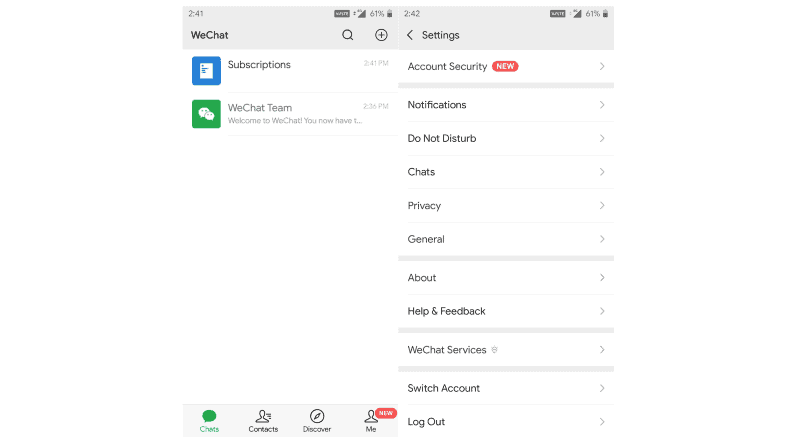The image comprises two screenshots taken on a mobile device, captured within the WeChat application.

In the first screenshot, the device’s time displays between 2:40 PM and 2:41 PM. The device is connected to a VPN, with full signal strength and the battery life at 61%. The top interface reveals the WeChat application name in black text, accompanied by a magnifying glass icon and a circle icon with a plus sign. A prominent blue button labeled "Subscriptions" is visible. Below, a message from the "WeChat Team" is partially visible with a green button, stating: "Welcome to the WeChat you now have..." The bottom navigation bar contains four icons: "Chats," "Contacts," "Discover," and "Me," with the "Me" icon appearing as newly designated.

The second screenshot, taken at 2:42 PM, showcases the settings menu of the WeChat app. The menu lists various options such as "Account Security" marked with a red notification bubble, followed by "Notifications," "Do Not Disturb," "Chats," "Privacy," "General," "About," "Help & Feedback," "WeChat Services," "Switch Account," and "Log Out."